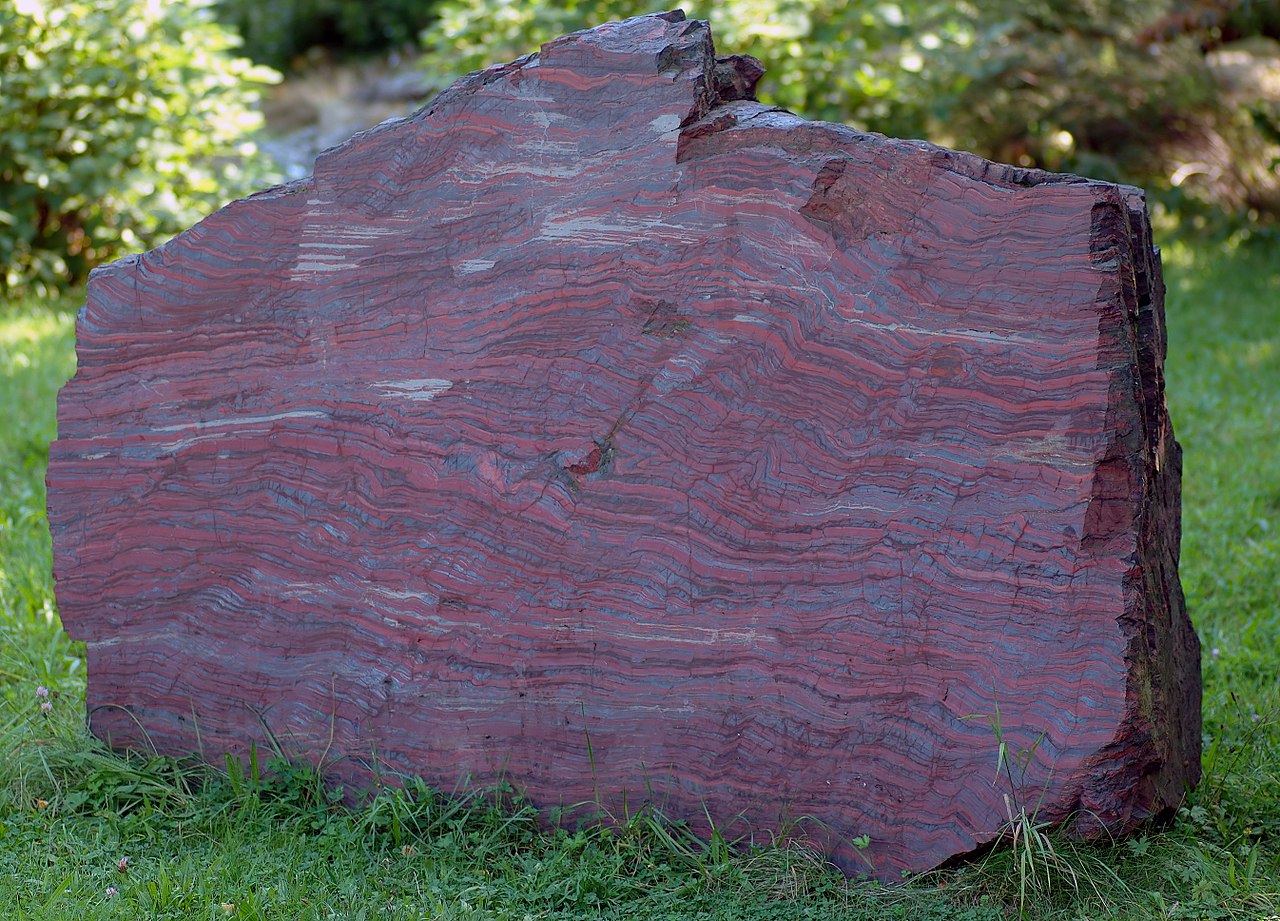The image captures a striking, unevenly-shaped rock with a jagged top that slopes downward, positioned prominently on a lush, green grassy surface. The rock exhibits a rich tapestry of colors, primarily dark red or burgundy interspersed with streaks of blue and white, giving it a foliated appearance with striations running horizontally through it. The rock's texture is rugged, featuring grooves and chips that add to its rugged charm. Surrounding the stone, the short, green grass is dotted with weeds, and in the background, a variety of bushes are bathed in sunlight, casting a yellowish hue on the leaves. A possible river glimmers faintly in the backdrop, hinting at the outdoor and daytime setting of this serene scene.